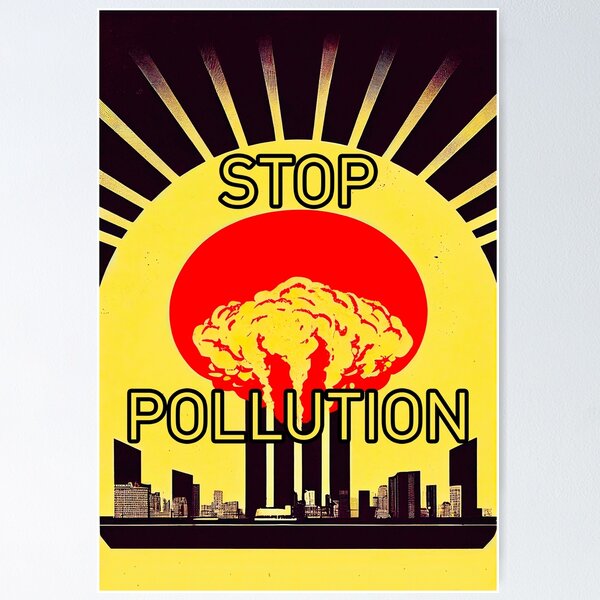The poster is a stark and eye-catching visual with a dominant black background. The focal point is a massive, stylistic yellow sun that occupies approximately 75% of the poster. Radiating from this sun are yellow rays that intensify the visual impact. The central imagery within the sun features a black cityscape of indistinct skyscrapers and buildings, suggesting urban sprawl. Prominently placed above and below the sun are the words "STOP POLLUTION," rendered in bold, yellow capital letters with black outlines for emphasis. Adding to the drama, a large, ominous red circle or mushroom cloud is positioned in the center, highlighted by white smokestacks billowing clouds of smoke. This powerful juxtaposition of bright yellow, stark black, and vivid red elements drives home the urgent environmental message of the poster.